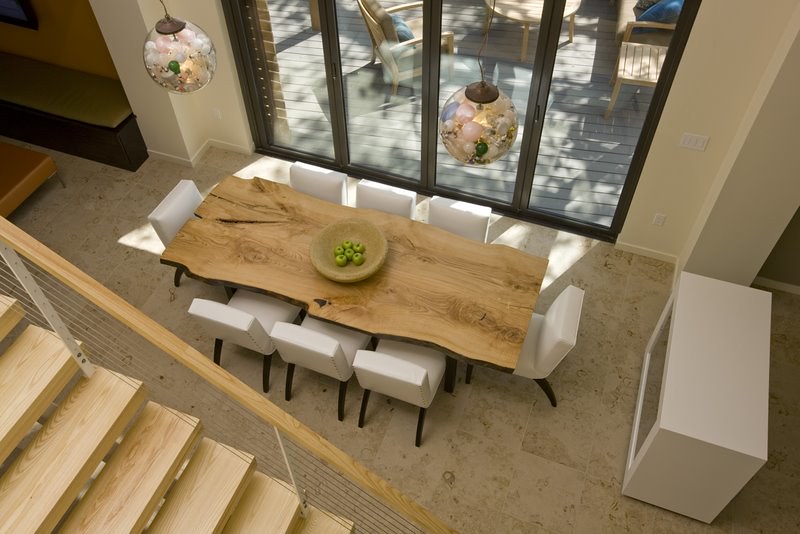In this detailed image taken from the top of a staircase during daytime, we get a comprehensive view of an indoor dining room and can glimpse the adjacent patio. The light wooden staircase with matching handrails descends to a floor that appears to be made of ceramic tiles. Central to the room is a long, natural wood table with a raw, untreated finish, a striking centerpiece that resembles a slab cut from the middle of a log. This table is surrounded by eight white, padded chairs with wooden legs—three on each side and one at each end.

Two distinctive lamps hanging from the ceiling stand out; they consist of glass orbs filled with small, colorful sphere-like elements in shades of white, pink, and green. The dining room also features a unique white hutch with brown drawers on the front, adding to the rustic yet elegant charm of the space.
 
A large, glass-paned door provides a view to the outside, revealing a wooden deck with ample seating—a continuation of the natural wood aesthetic present inside. The patio set includes wooden chairs and a table, creating a seamless flow between the indoor and outdoor living areas. On the right side of the dining room, a white table set against the wall adds to the room's functionality. Additionally, there is a wooden bowl filled with green apples adorning the center of the dining table. This beautiful dining space combines raw wooden elements with modern, clean lines for a welcoming and charming atmosphere.